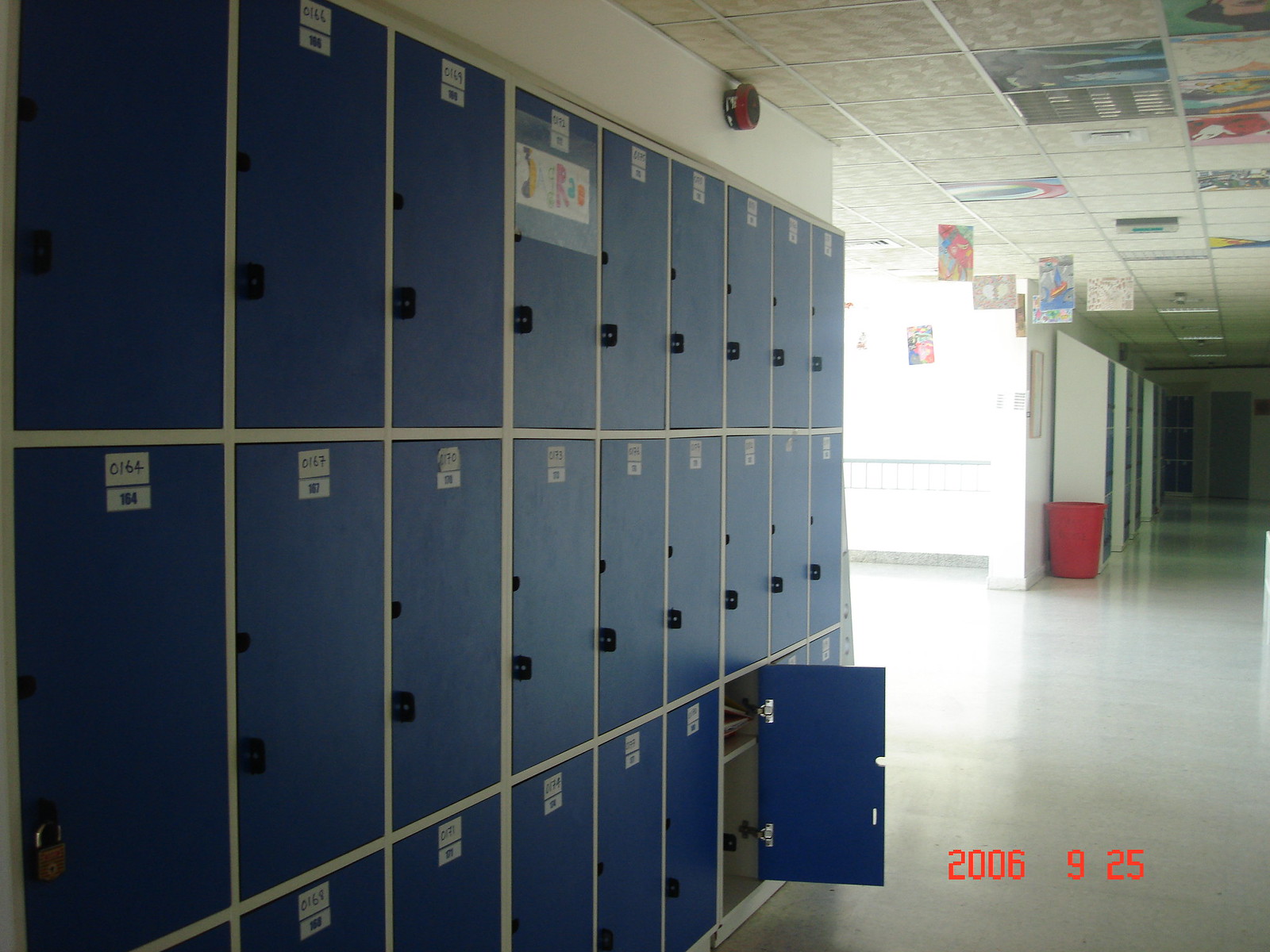This photo captures the interior of a school building, specifically a long hallway. The flooring is white vinyl, complemented by white walls. Lining the hallway on the left side are three rows of blue square lockers, each marked with numbers. Among these lockers, one has a lock, and another stands open, while the rest are closed without locks. Above the lockers, a red fire alarm is mounted on the wall. The ceiling features vents for heating and air conditioning, accompanied by some papers and a paper with "2006-925" written on it hanging from and attached to the ceiling. Additionally, a red garbage can is situated farther down the hallway. The end of the hallway is quite dark, contrasting with the bright light spilling in from an adjacent hallway or a large window near the entrance, highlighting the white walls and intensifying the brightness of the immediate space.